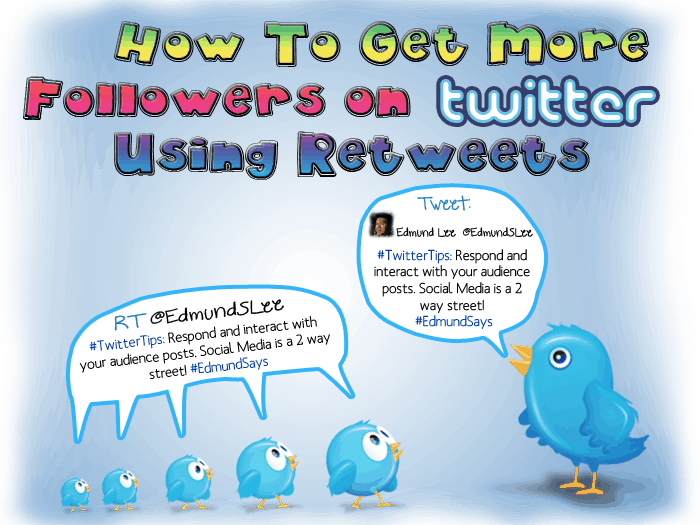The image is an informational comic with a casual design. The background features a light blue pastel tone. The top portion of the comic has three rows of text. The first row reads "How to Get More" in green block letters with darker green engravings. Below, the second row contains "Followers on" in red or maroon text, followed by "Twitter" aligned to the right, styled to resemble the Twitter logo. The third row says "Using Retweet," displayed in metallic blue text.

In the bottom right corner, there is a larger blue bird with a speech bubble that reads "Tweet Edmond S. Lee." The bird also includes the hashtag "#TwitterTips." 

Adjacent to the larger bird, the caption emphasizes, "Respond and interact with your audience. Social media is a two-way street," with the number two represented numerically.

To the left, there are five smaller birds, arranged in a gradient with the largest on the right. Each bird is depicted with a speech bubble saying "RT." The text nearby also reads "Edmond S. Lee," followed by the hashtag "#TwitterTips." Additionally, another caption reiterates "Respond and interact with your audience. Social media is a two-way street," finalized with the hashtag "#EdmondSays."